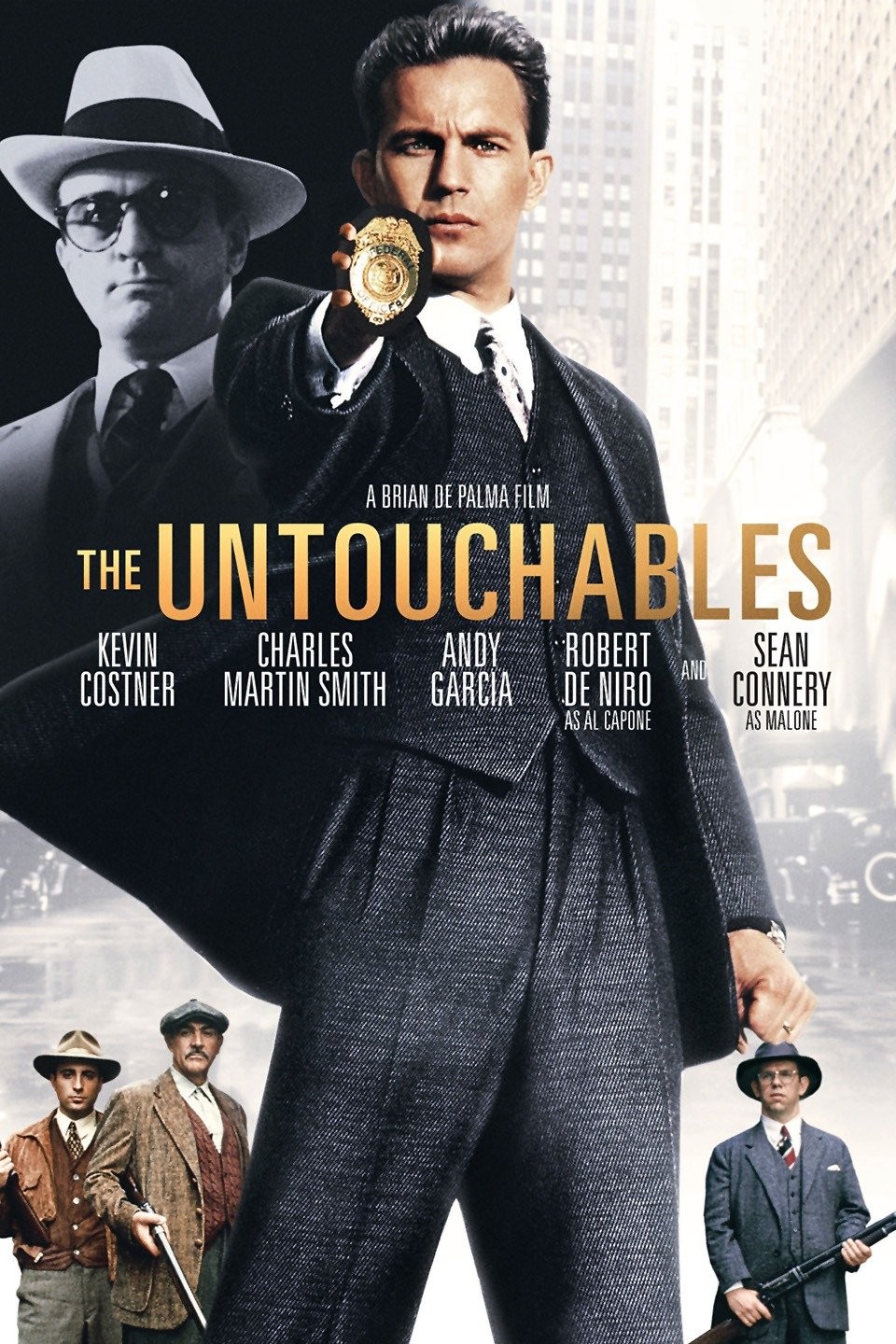The poster advertisement for the movie "The Untouchables" vividly captures a dramatic and intense moment. At the center stands Kevin Costner, holding out a policeman's badge with a stern and unwavering look on his face, dressed in a sharp black suit and white shirt. To his upper left, a black and white photograph of Robert De Niro as Al Capone, wearing a white fedora and glasses, looms ominously. The bottom left of the poster features small, colored images of two men, both sporting fedoras, while on the bottom right, another man grasps a shotgun, donning a gray hat. Across the center, bold text proclaims it as "A Brian De Palma Film, The Untouchables," followed by the names of the star-studded cast: Kevin Costner, Charles Martin Smith, Andy Garcia, Robert De Niro as Al Capone, and Sean Connery as Malone. The backdrop features a hazy, almost dream-like depiction of a city with towering buildings, and towards the bottom, the street is lined with black cars, adding a touch of historical authenticity. This combination of vibrant and monochromatic elements along with the cast's intense gazes create a striking and memorable promotional image.